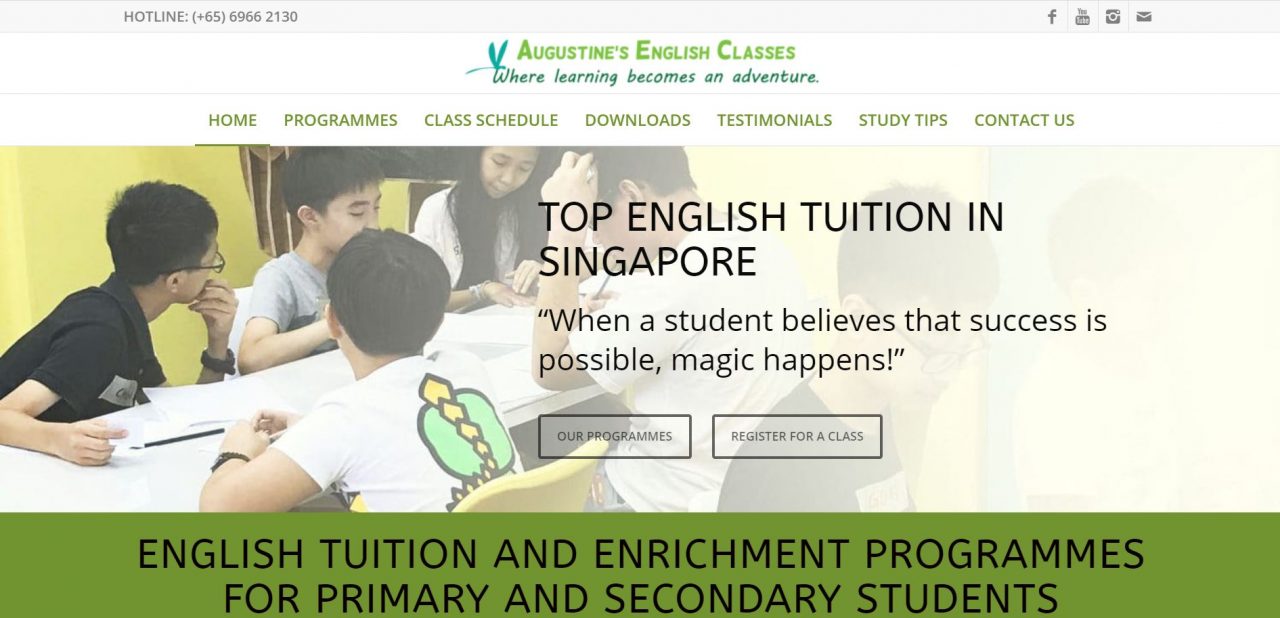Screenshot of a Website on an Apple Computer:

The screenshot captures a website, likely viewed on an Apple computer. The taskbar at the top of the screen is grey and contains important navigation and contact information. At the top-left corner, the word "Hotline" is displayed, followed by the phone number "(+65) 69662130." Moving towards the right-hand side of the taskbar, there are icons for social media platforms and other links, including Facebook, YouTube, email, and an unidentified site.

Below the grey taskbar, the header of the website features a white background with the text "Augustine's English Classes" accented by a teal element before the word "Augustine's." Beneath this, in blue text, is the tagline "Where Learning Becomes an Adventure." The navigation tabs for the website are located underneath this header in a grey bar, including options such as Home, Programs, Class Schedule, Downloads, Testimonials, Study Tips, and Contact Us.

The main content area displays a large photograph that spans the entire width of the site. On the left side of the image, students are seated at tables with books in front of them; they are set against a backdrop of a yellow wall and a bookcase. The image fades to a cream color as it approaches the right side of the page. Superimposed on the photograph is the text "Top English Tuition in Singapore" and the motivational statement "When a student believes that success is possible, magic happens."

Below the photograph are two prominently displayed blocks for "Our Programs" and "Register for a Class." At the bottom of the screenshot, there is a deep apple green bar that runs across the entire width of the website, featuring black text that reads "English Tuition and Enrichment Programs for Primary and Secondary Students."